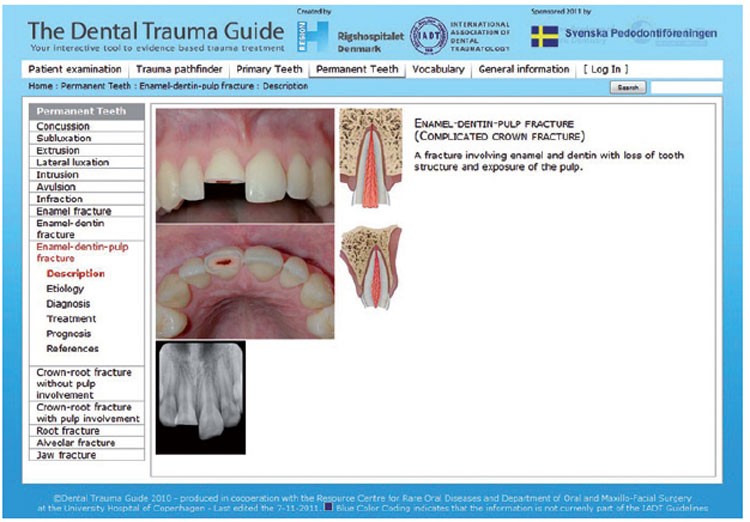This detailed screenshot from the Dental Trauma Guide website features a prominent header in the upper left corner identifying the site. The guide is co-sponsored by the International Association of Dental Traumatology and Rigshospitalet, Denmark, with visual symbols including a purple emblem and a dark blue flag with a yellow cross. The page includes various navigational tabs such as Patient Examination, Trauma Pathfinder, Primary Teeth, Permanent Teeth, Vocabulary, General Information, and Login. These tabs are designed to help users traverse through different sections of dental trauma information.

The main content area displays two high-resolution photographs of a broken tooth from different angles—one frontal view showing the damage directly and one underside view revealing the exposed red pulp. Additionally, there is an illustrative diagram explaining the condition known as an enamel-dentin pulp fracture, also termed as a complicated crown fracture. This detailed diagram highlights the fracture involving enamel and dentin with loss of tooth structure and pulp exposure. Beneath these photographs, an x-ray image provides further visual context of the tooth's internal damage. On the left side, a comprehensive list categorizes various types of dental trauma and fractures, ensuring a wide range of information is accessible for both educational and clinical reference.